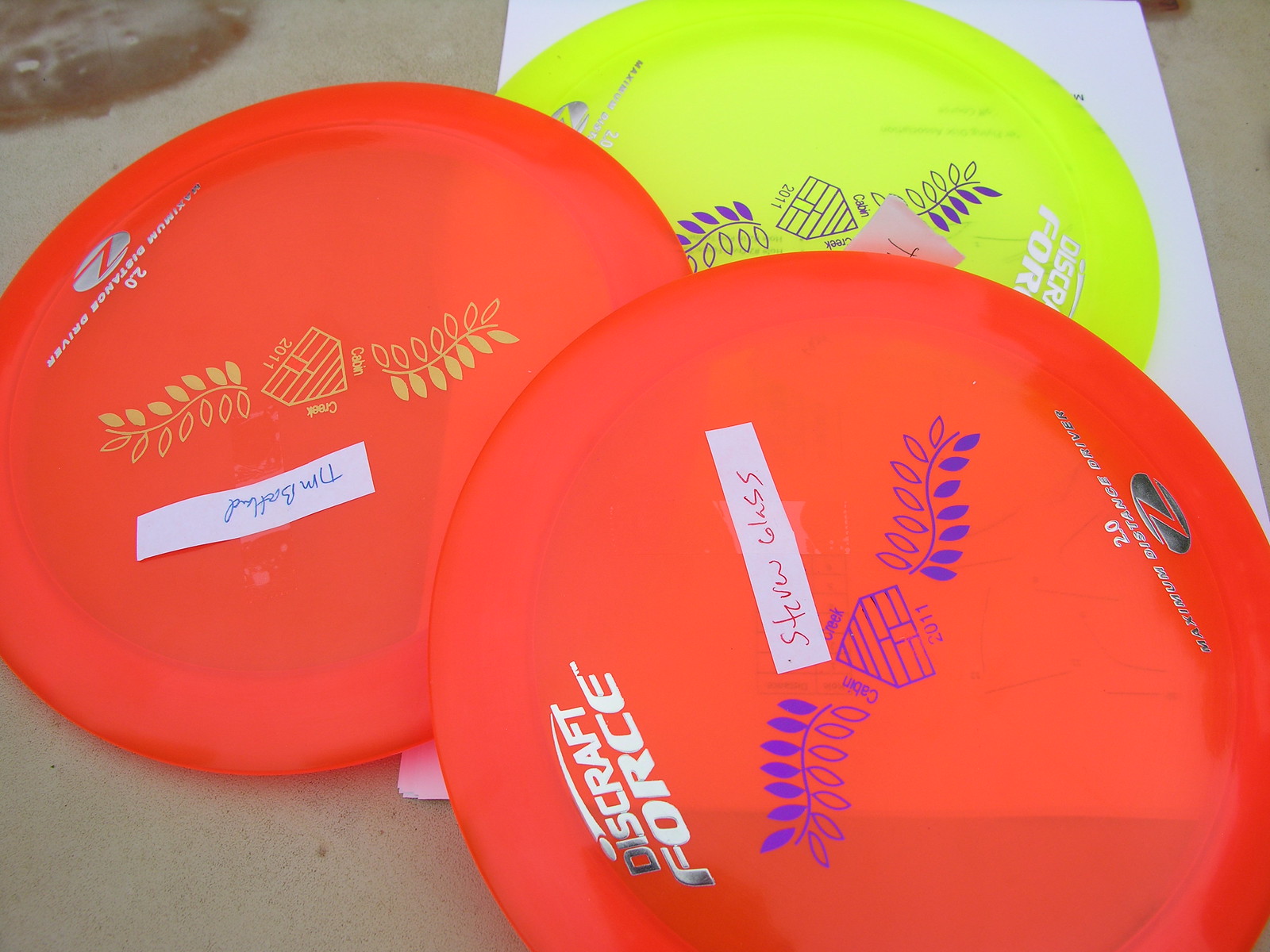The color photograph presents a detailed close-up of three frisbees stacked on top of each other and resting on a table, under which lies a long white piece of paper. The frisbee at the bottom is an electric, high-visibility, neon yellowish-green color, adorned with purple leaves and outlines of uncolored leaves, forming a graphic that includes a logo of a cabin or beehive with an inscription of "Creek" and the number "2011." Above it, there are two bright orange frisbees, each featuring a similar design with blue designs of leaves and markings and inscribed with "Discraft Force" in white lettering. Both orange frisbees have white tape affixed to them, marked with names in ballpoint pen: one tape reads "Steve Glass," while the other, oriented upside-down, appears to say "Tim Somebody."